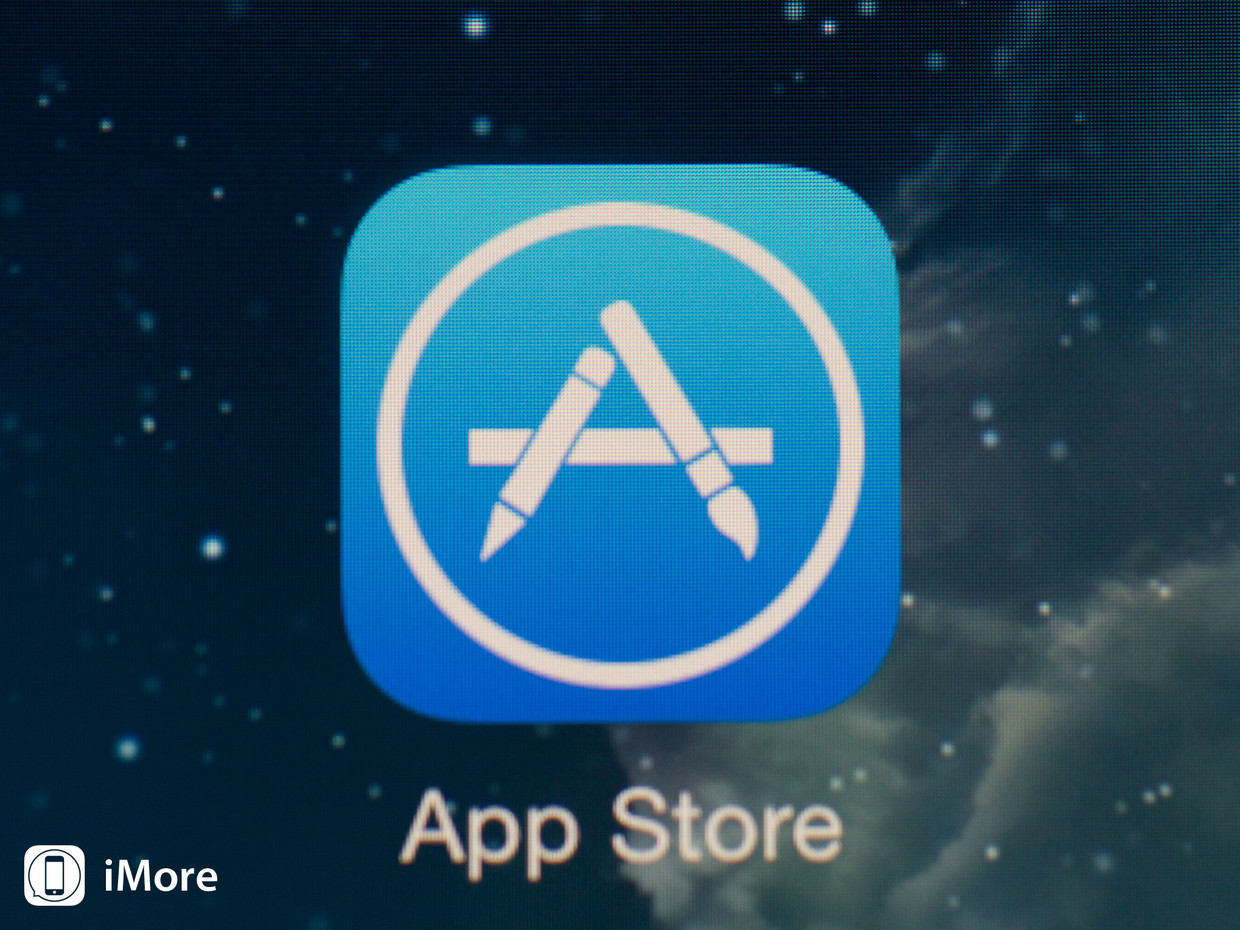This image captures an Apple device displaying the App Store logo prominently at its center. The App Store emblem is a blue rounded square with a gradient, transitioning from light blue at the top to darker blue at the bottom. Inside the square sits a white circle hosting the App Store's distinctive "A" symbol, artfully formed by a stylized pen, pencil, and horizontal line. Below the logo, the words "App Store" are inscribed in clean, white text. The bottom-right corner of the image features the iMore logo, consisting of the word "iMore" and an adjacent white square with a phone icon in the center, representing the branding of the image source. The overall visual is slightly fuzzy, suggesting it is a physical photograph of the device rather than a screenshot. The backdrop surrounding the App Store logo and text depicts a serene, dark blue starry night sky adorned with delicate clouds and twinkling stars, enhancing the allure of this Apple device's display.